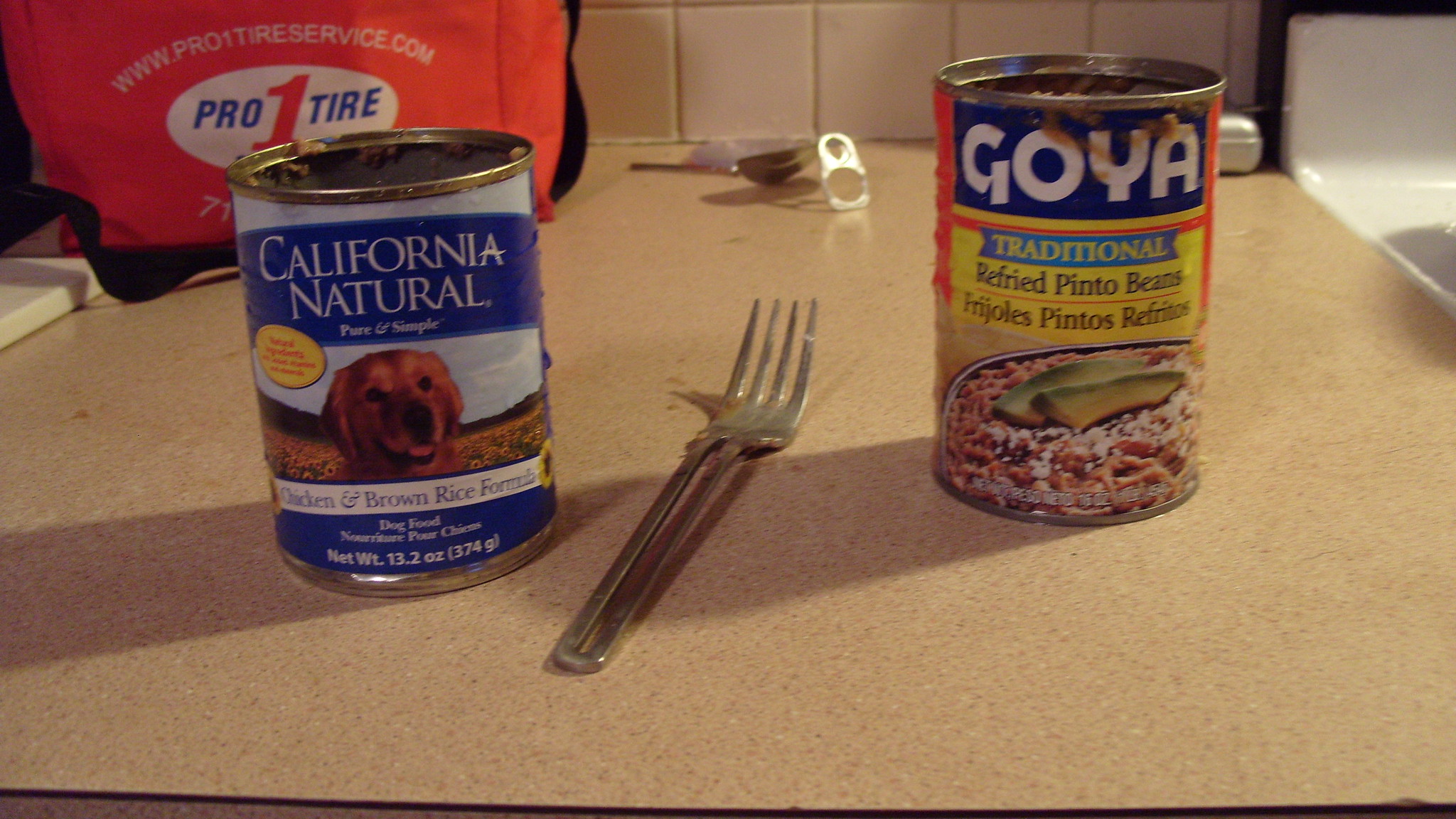In this color photograph taken indoors in landscape mode, two cans of food are displayed on a brown counter. Positioned between them is a shiny metal fork. The can on the right, boasting the brand name "Goya," contains traditional refried pinto beans and is open. Its label features an appetizing image of refried beans garnished with two slices of avocado and a sprinkling of crumbled white cheese. The can on the left, labeled "California Natural Chicken and Brown Rice Formula," is also open and intended for dog food. Its label includes a photo of a brown dog. It appears that someone has potentially mixed the contents of the dog food with the pinto beans, suggesting an unexpected culinary combination.